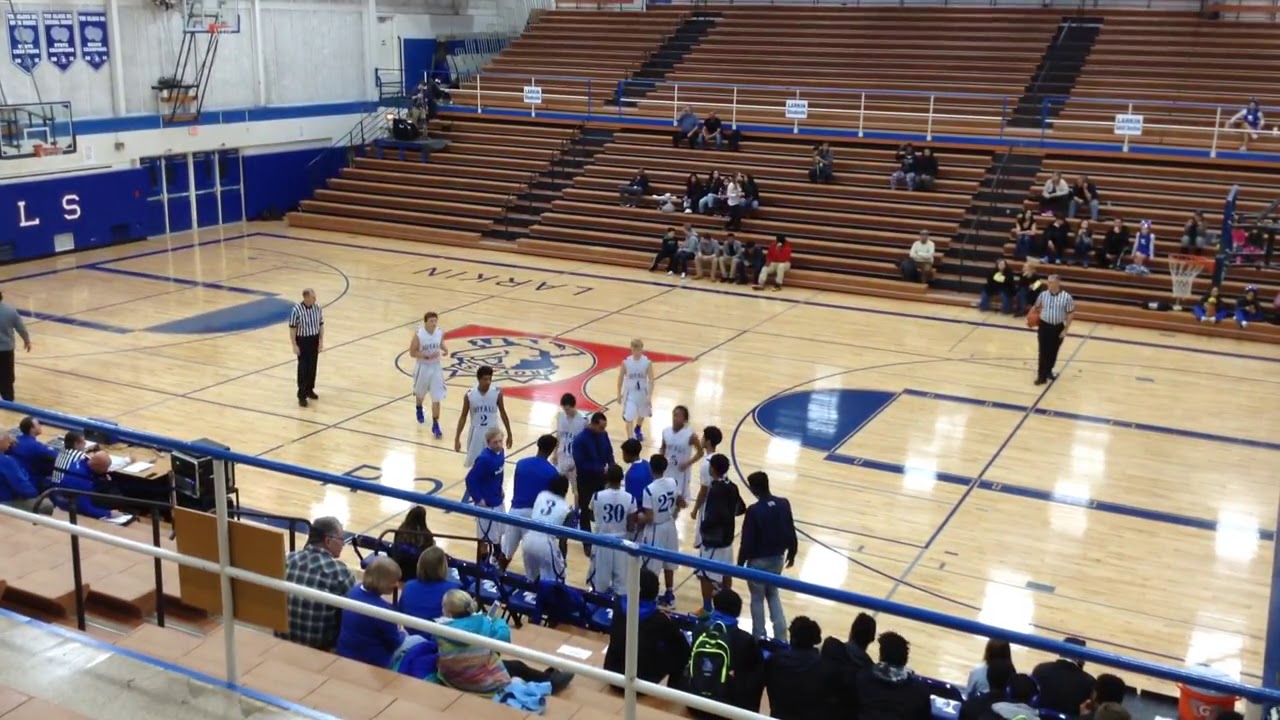The image captures an indoor basketball court with shiny light wood flooring, marked with blue and red designs. The vantage point is from the bleachers, providing a slightly elevated, downward view. In the center of the court, basketball players in white and blue uniforms are gathered around their coaches. Additionally, several individuals in blue shirts, including dress shirts, are also seen among the players. Two referees are visible: one on the left side of the court and another on the right, holding a basketball. 

The scene includes a crowd, primarily filling the bottom half of both sets of bleachers. The court features two visible basketball goals and a partially visible red and blue logo in the center, with the word "Larkin" noted on the right side of the court. The area is brightly lit, with reflections from the overhead lights shimmering on the polished court surface.